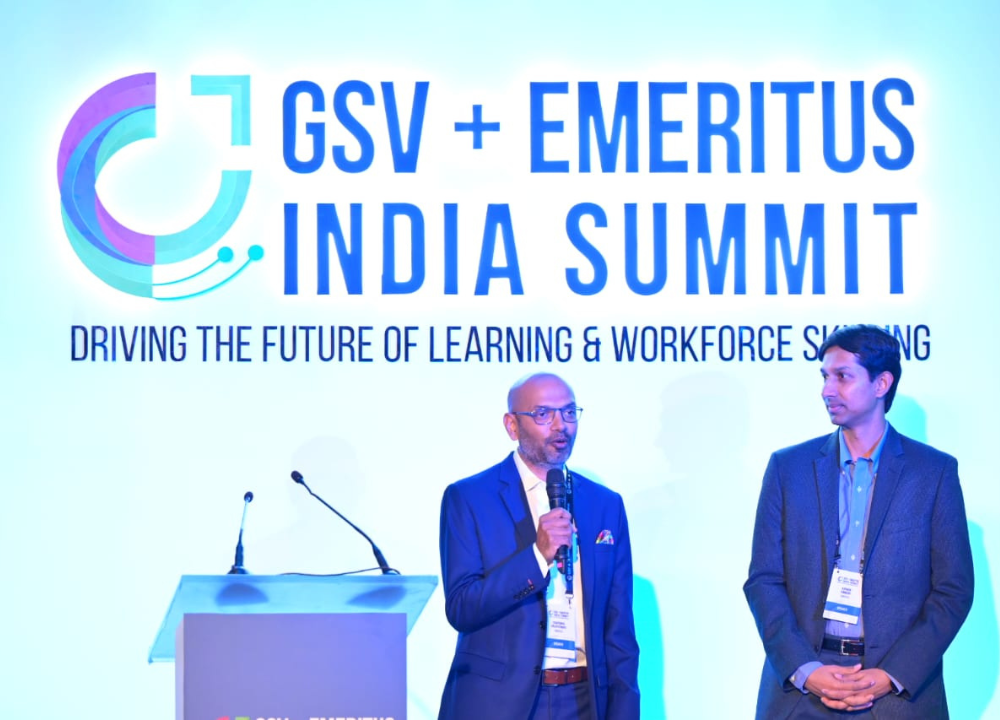This indoor photograph captures a business conference, specifically the GSV + Emeritus India Summit, focused on "driving the future of learning and workforce." The background features a light blue backdrop with purple, blue, and green logos, and prominently displays the summit's title in blue text. Centered in the image, a dark-skinned man of Indian descent stands to the right of a white podium equipped with two microphones. He is holding a black microphone and addressing the audience. He sports a blue sport coat, white business shirt, brown belt, and blue pants, complemented by a lanyard and name tag. He is bald with glasses and a light beard. To his right, another man, slightly taller with dark hair, is dressed in a blue suit and shirt. He also wears a lanyard and looks attentively at the speaking gentleman.